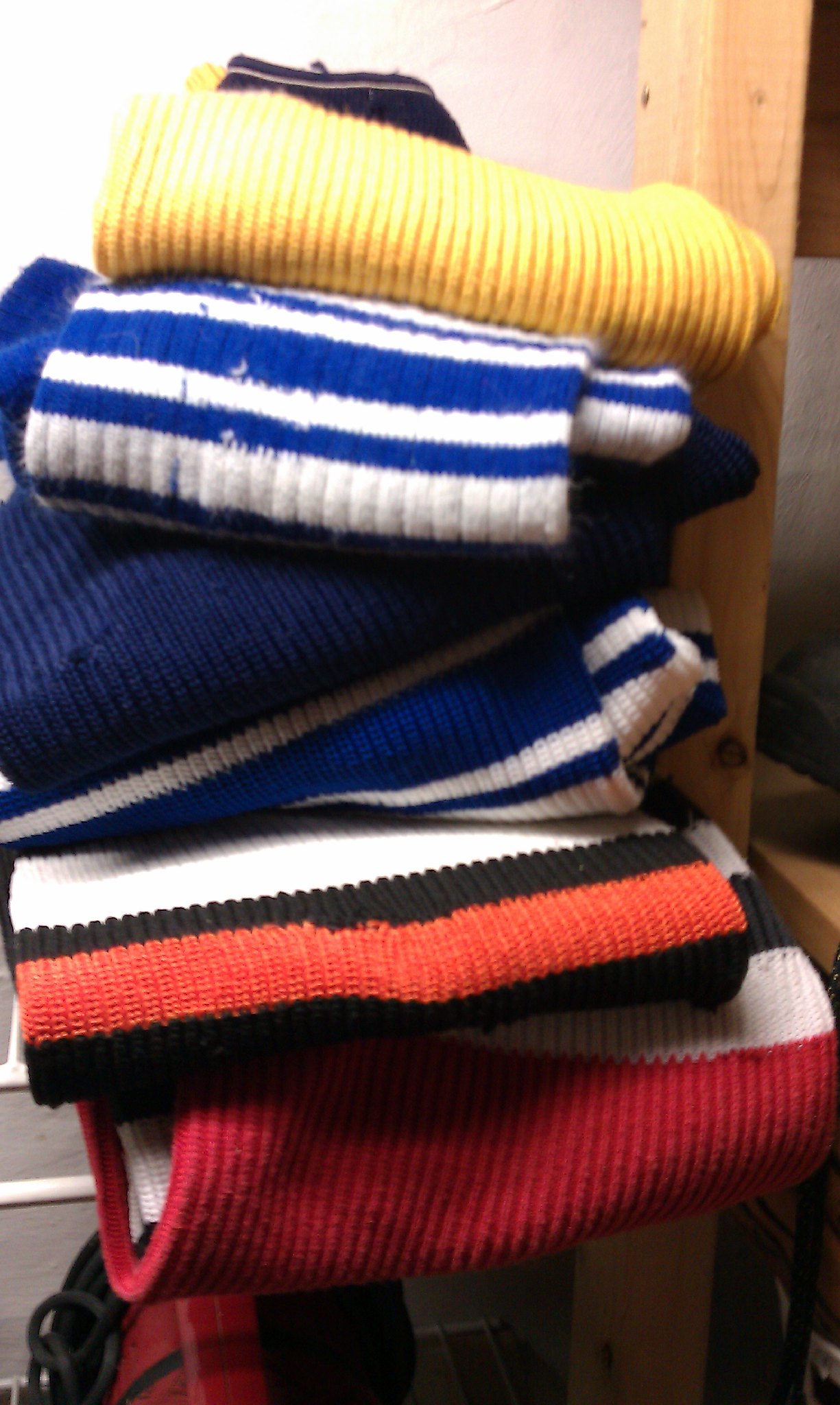The image depicts a neatly stacked assortment of knit sweaters, situated on a white metal shelf likely set in a closet. The top sweater in the stack is a yellow knit with a brown collar. Beneath it lies a white and blue horizontally striped sweater, followed by a navy blue knit sweater with a small hole. Below that, another striped sweater in navy blue and white is visible. The next item is a visually distinct knit sweater adorned with broad stripes of white, brown, and orange. Finally, at the bottom of the stack is a sweater with red, brown, and white stripes. The shelf, with its white metal structure, appears against a background that includes wood trimming towards the right, and possibly a pine wood shelf seen behind the sweaters. The image also hints at the lower part of the shelf where there appears to be a red vacuum cleaner with a black cord wrapped around it. The sweaters, seemingly sized for children around ten years old, lend the image a cozy, organized feel typical of cooler weather attire.